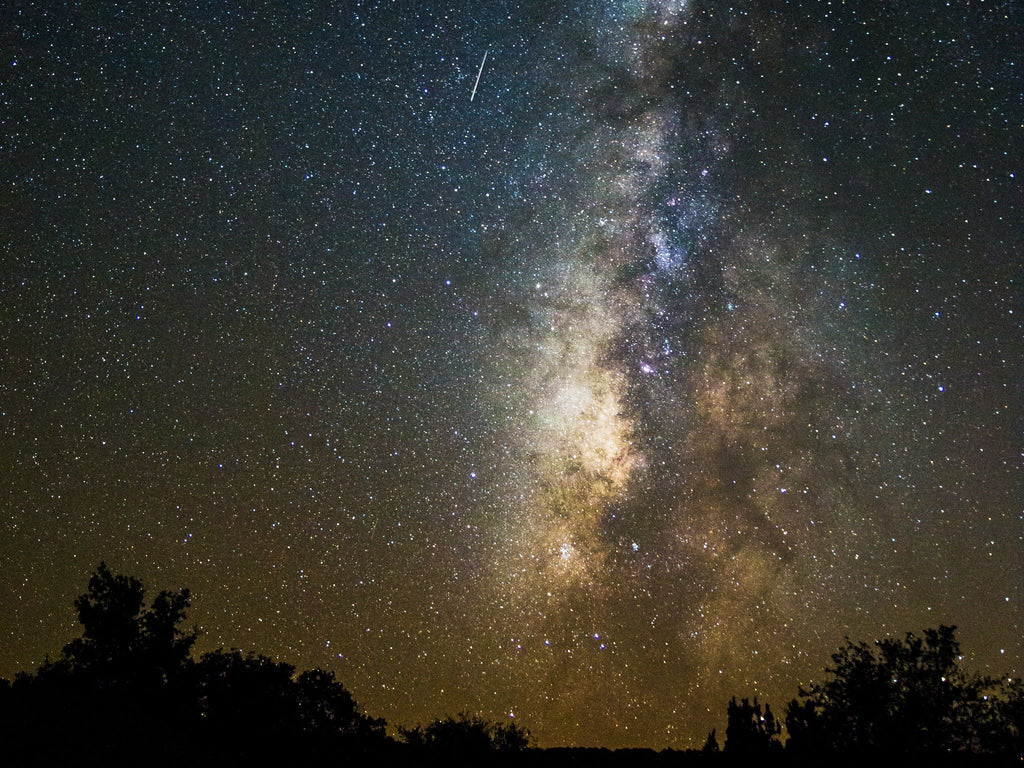This photograph captures a stunning night sky, filled with thousands of stars of varying colors, including blue, yellow, and even reddish hues. The top of the image showcases a purplish sky that transitions into a yellowish-gray toward the bottom. Dominating the center is a striking vertical band resembling a nebula or possibly a group of galaxies, filled with clumps of white, light blue, and gray colors. This band stretches from the top almost to the bottom of the image, branching out into intricate patterns. A shooting star is visible in the top center-left portion of the sky, adding to the celestial wonder. At the bottom of the photo, silhouetted against the expansive sky, are a series of trees. These trees range from tall on the left, tapering down to shorter, bush-like forms in the middle, and then growing taller again towards the right edge. The outline of the trees, with their varying heights and dark silhouette, contrasts beautifully with the luminous and colorful night sky above.